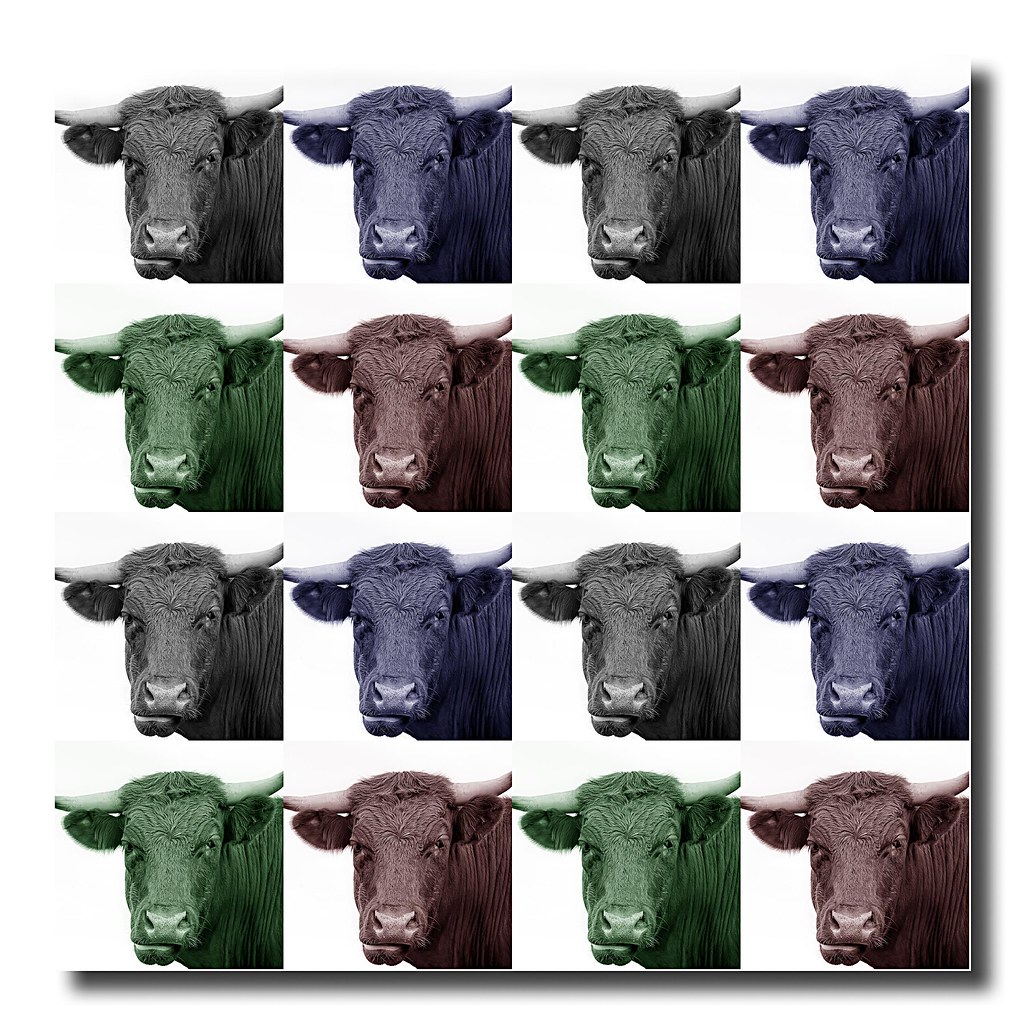This image is an artistic rendering designed as wall art, featuring a grid of 16 identical pictures of a bull arranged in four rows and four columns. Each depiction of the bull is in a different color, creating a distinctive pattern: the first and third rows alternate between black and purple bulls from left to right, while the second and fourth rows alternate between green and red bulls. The colors repeat vertically as well: black and green bulls alternate in the first column, followed by purple and red in the second. The bull's face, characterized by its outward-pointing horns, prominent eyes, and side-protruding ears, is the focal point of each picture, though a small portion of the body is also visible. Additionally, each image has white shadows on two of its edges, giving it a floating effect. This art piece, reminiscent of something you might find in a modern home goods store like Target, uses color variations to add a playful and visually captivating element to the composition.